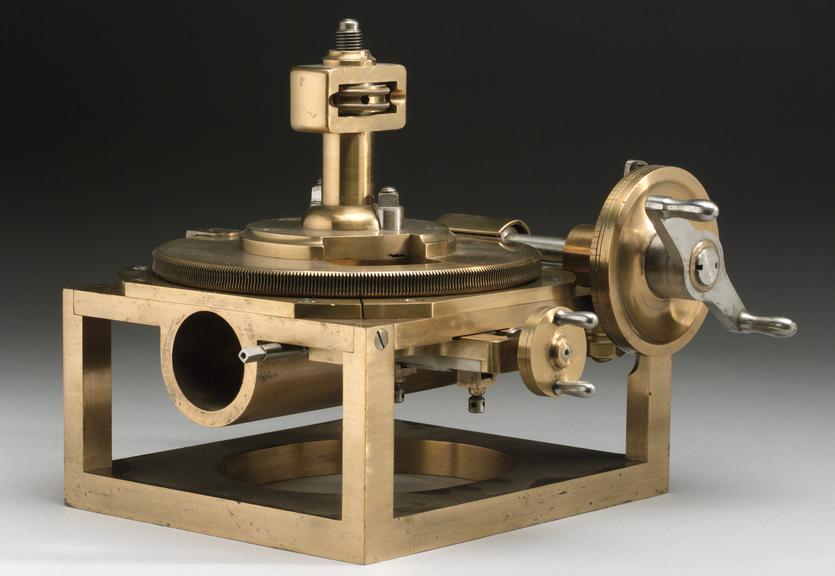This photographic image, set in an indoor environment, showcases a complex piece of gold-colored machinery with chrome accents. The machinery sits on a sturdy, square metal base elegantly shaded from light gray to dark at the top. Central to the device is a fishing rod-like knob attached to a rod, which connects to a cylindrical hub and gear system. On this gear, two vertical posts support a small enclosure housing another gear.

The structure includes several hand-crank mechanisms resembling those found on a lathe, suggesting a function related to precise machining. The top displays a flywheel with gear-edged rims, connected vertically to a silver shaft resembling a pulley within an enclosure. The base also features a hollow cylinder and additional adjustment wheels, emphasizing its intricate, mechanical nature.

Surrounded by a four-sided rectangular frame forming a transparent square, the machine's artistic layout stands out against a background that gradients from black at the top through gray to white at the bottom. The overall design hints at both functionality and careful craftsmanship, although its specific purpose remains an enigma. The image contains no text or human elements, focusing solely on this enigmatic and meticulously constructed device.